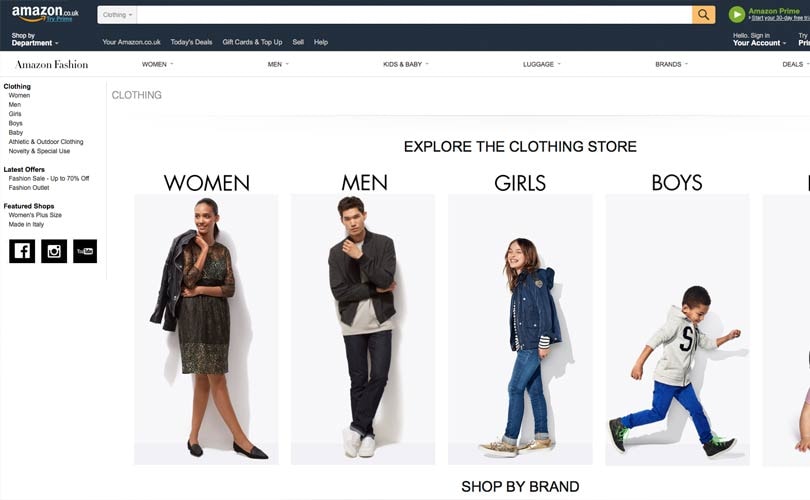The screenshot captures a section of the Amazon.com website, specifically the Amazon Fashion tab. The image is cropped, with the right side cut off. At the center of the page, there are four prominent thumbnails labeled "Women," "Men," "Girls," and "Boys." Each category showcases a large image of a model wearing an outfit relevant to that category. Directly beneath these thumbnails, a section titled "Shop by Brand" is centered.

On the right side of the screenshot, a column displays various categories. The first category is "Clothing," which includes several subcategories underneath it. The second category is "Latest Offers," followed by "Featured Shops" as the third category. Below the "Featured Shops" section, there are three social media icons in square boxes representing Facebook, Instagram, and Reddit.

Additionally, there are navigation categories across the top of the webpage, each with drop-down menus. These categories include "Women," "Men," "Kids & Baby," "Luggage," "Brands," and "Deals."